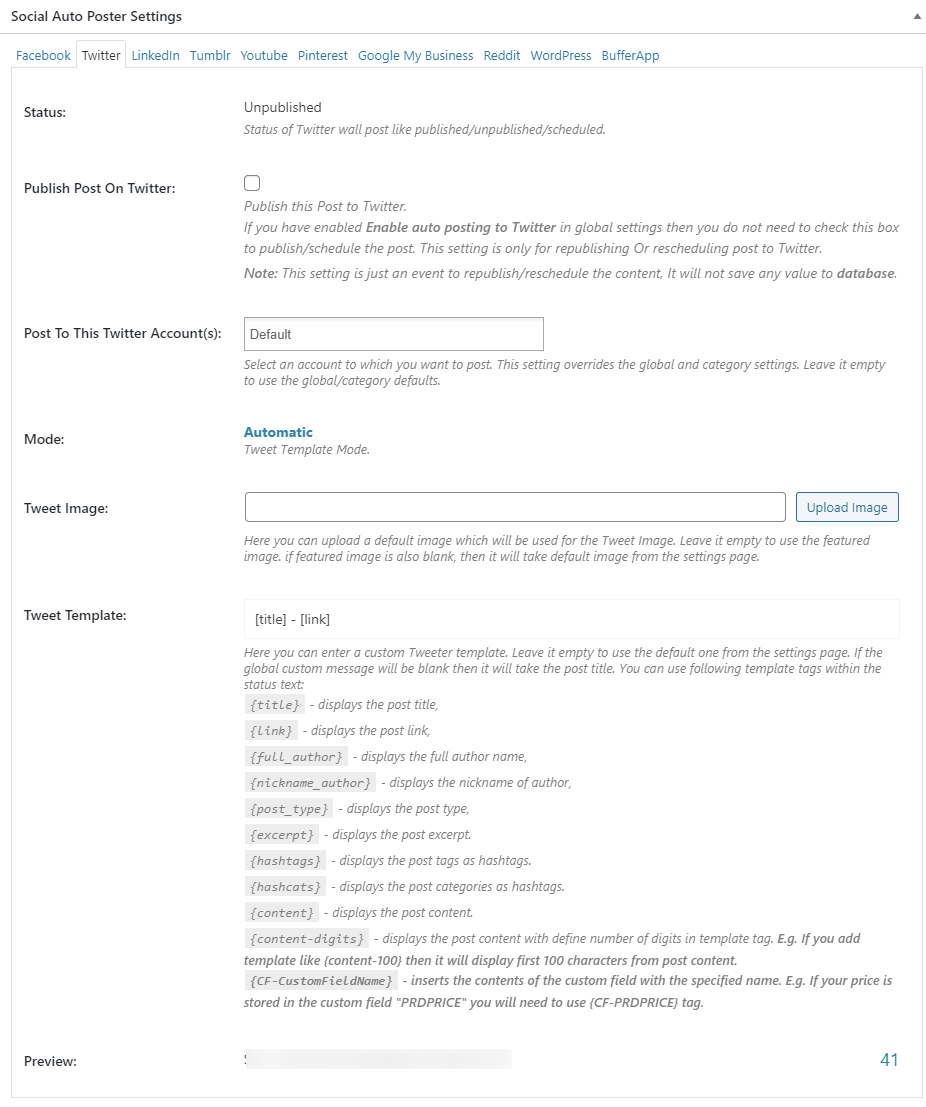This image is a detailed screenshot from a website's settings interface for a social media auto-poster tool. At the top of the interface, there's a header in black text reading "Social Auto Poster Settings." Below the header is a thin, light gray line separating it from the next section. 

The next portion features a list of social media platforms, each named in blue text, except for Twitter, which is in gray. The platforms are listed in the following order: Facebook, Twitter, LinkedIn, Tumblr, YouTube, Pinterest, Google, Google My Business, Reddit, WordPress, and Buffer App.

Beneath this list is a larger square section containing additional options for Twitter specifically. In this section, "Status: Unpublished" is indicated in black text. Below this, a checkbox option labeled "Publish post on Twitter" is present, accompanied by an instruction that reads, "If you have enabled auto posting to Twitter in global settings, then you do not need to check this box to publish."

Further options include "Schedule this post," "Post to Twitter accounts," and a "Default mode: Automatic" option highlighted in blue text. Additional settings here are "Tweet template mode," "Tweet image" with an explanation that users can upload a default image for the tweet, or leave it empty to use the featured image, and the label "Tweet template," followed by a "Preview" option.